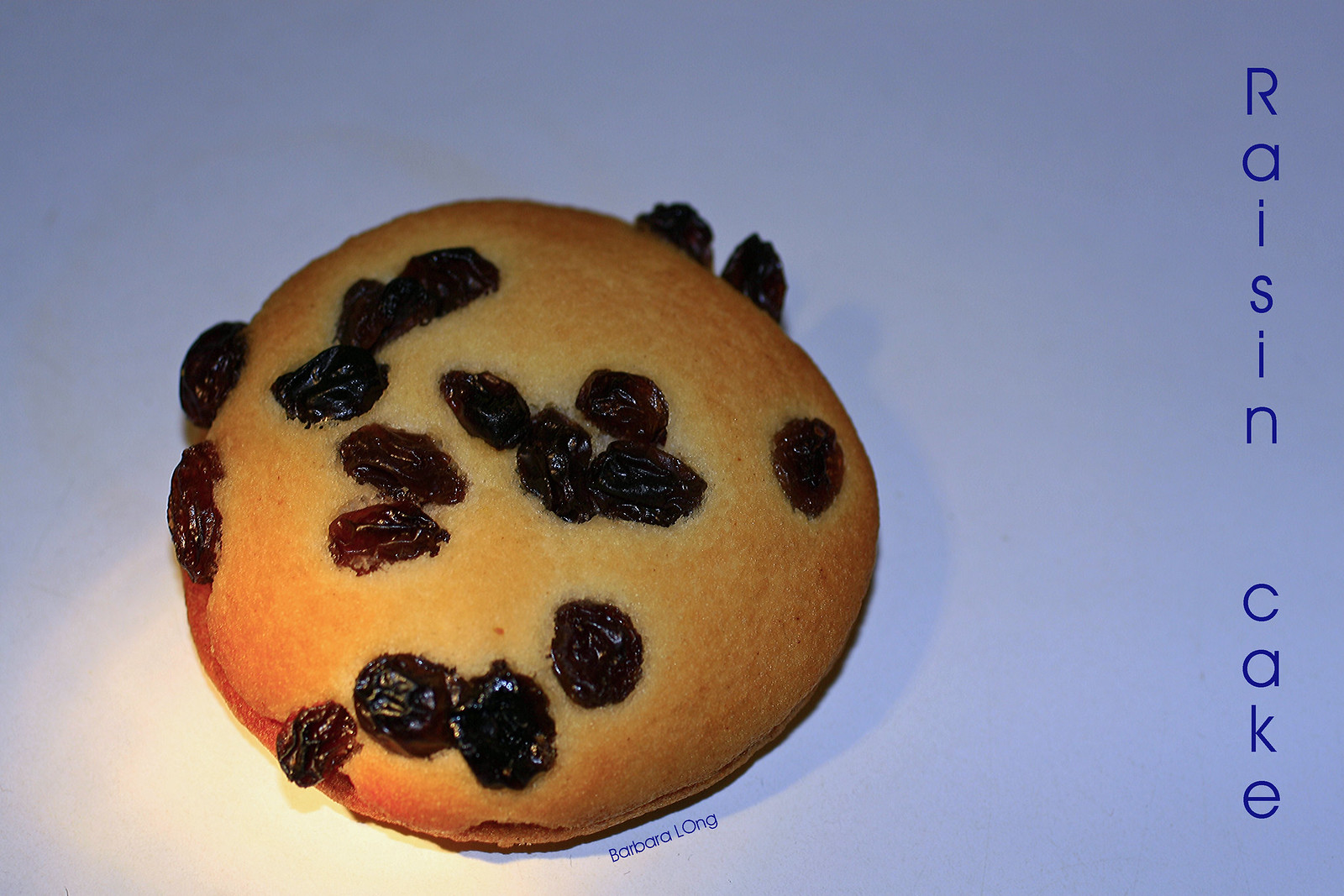This image prominently features a circular raisin cake set against a purplish-white background. The cake has a light brown, tan body, generously topped with sixteen evenly distributed black raisins. Specifically, nine raisins are near the center, with six encircling the middle area, and the remaining five strategically placed around the edge at various clock positions. To the right, in vertically aligned dark blue text, are the words "Raisin Cake." Below the cake, the name "Barbara Long" is written, with a distinctive capitalized "O" in "Long." This detailed arrangement and textual elements suggest the image might be digitally enhanced for visual clarity.